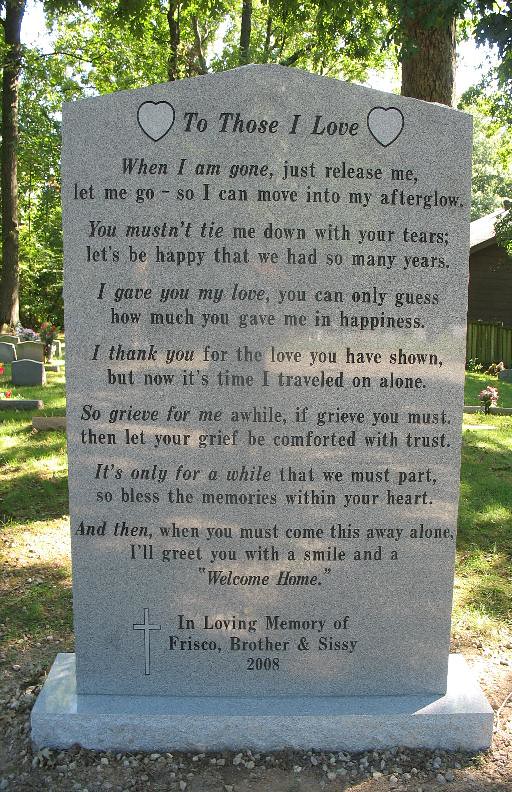This photograph captures a tall headstone in a graveyard with intricate engravings that convey a heartfelt message. At the top of the headstone, flanked by hearts on either side, is the heading, "To Those I Love." Below this, an elegant message is inscribed, encompassing thoughts of love, grief, and the eventual reunion in the afterlife. The inscription reads:

"When I am gone, just release me, let me go, so I can move into my afterglow. You mustn't tie me down with your tears; let's be happy that we had so many years. I gave you my love; you can only guess how much you gave me in happiness. I thank you for the love you have shown, but now it's time I traveled on alone. So grieve for me a while, if grieve you must, then let your grief be comforted with trust. It's only for a while that we must part, so bless the memories within your heart. And then, when you come this way alone, I'll greet you with a smile and a welcome home."

At the bottom, between a small engraved cross, it reads, "In loving memory of Frisco, brother and sissy, 2008." This poignant tribute captures the enduring connection between Frisco and his loved ones, offering solace and hope with the promise of a future reunion.